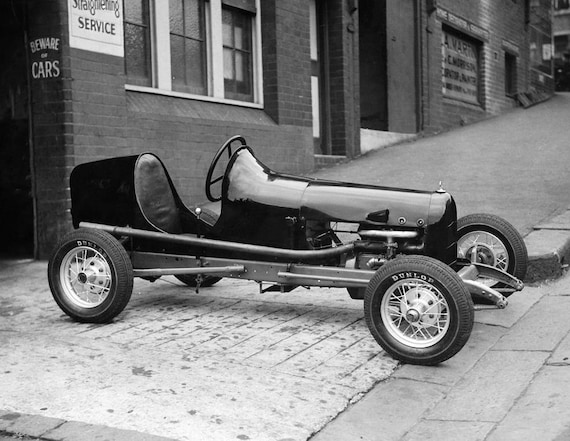This black and white photograph showcases a vintage midget race car, likely from the 1930s to 1950s, parked in a narrow downtown area. The sleek, canoe-shaped vehicle, designed for a single driver, features a shiny black metal body and low-to-the-ground Dunlop tires, two in the front and two in the back. Despite its racing nature, the seat offers minimal comfort with a slightly cushioned backing. Positioned sideways on a sidewalk, the car is captured against a backdrop of street buildings, including signs that read "service" and "beware of cars." This evocative image highlights the historic charm and distinctive design of early race cars.